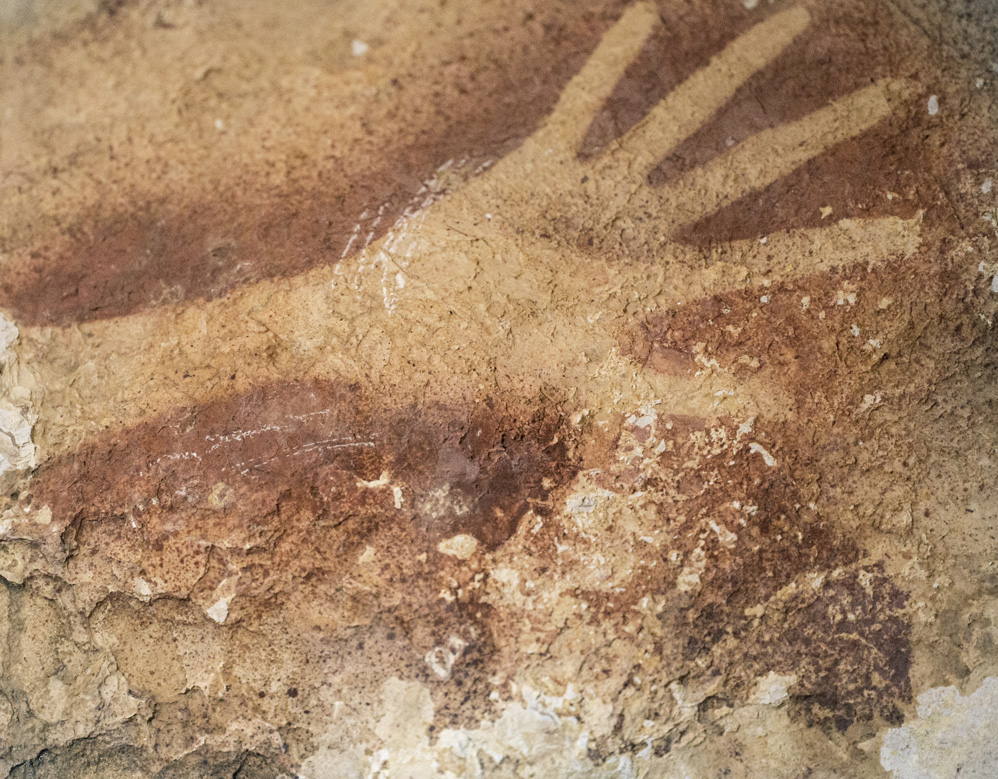The image depicts a weathered rock wall with a prominently imprinted or painted human hand in the center. The rough, grainy texture of the rock, which appears to be a mix of tan, gray, and dark brown, gives it an aged, almost prehistoric look, similar to chipped sandstone. The handprint itself is a striking light tan color with a dark brown outline tracing the edges of the fingers, wrist, and forearm, making it stand out vividly against the mottled surface. The hand features elongated fingers, a relatively large palm, and a slender wrist extending partway up the forearm. The surrounding area of the rock shows different hues, with hints of white and darker shades intermingling with the predominant earth tones, adding to the impression of a surface that has been shaped by time and elements.